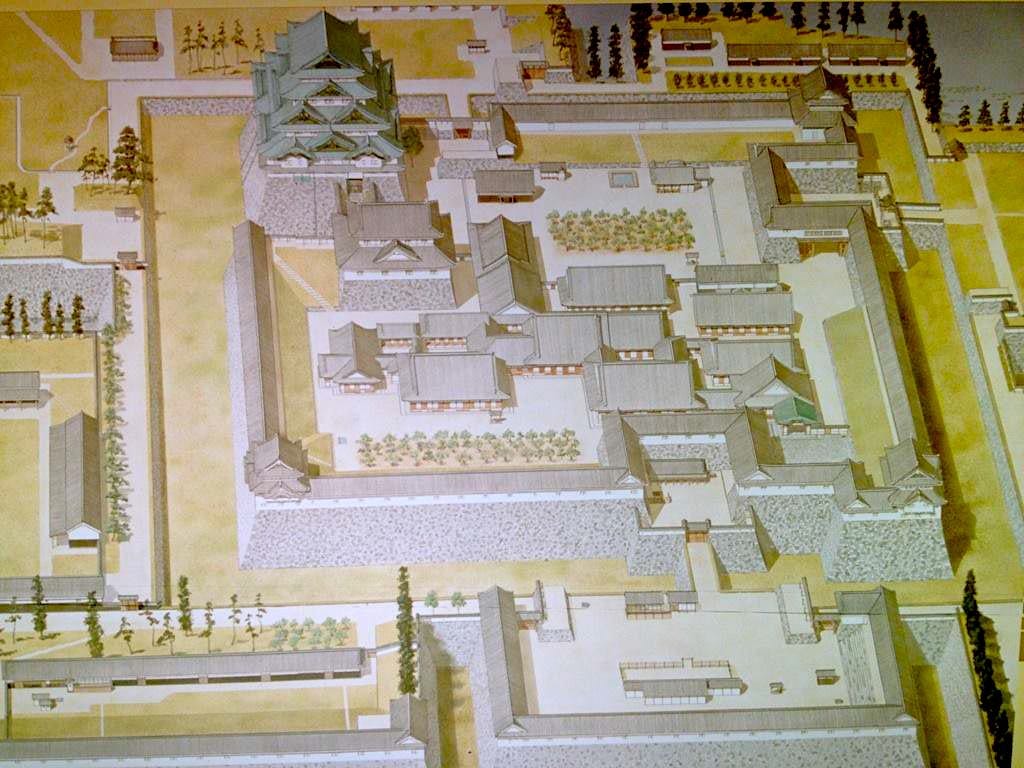The image appears to be a highly detailed three-dimensional diorama or architectural model depicting a large complex. It showcases a bird's-eye view, possibly of a feudal Japanese castle or a new factory or plant design. The setting includes numerous gray buildings and intricate pathways marked in yellow, with an abundance of green trees lining the streets and roads. The inner area features what seems to be a significant tower or palace, green-roofed and surrounded by smaller structures, all placed within a thoughtfully designed layout including a moat and several entrance points. This could serve as a professional architectural rendering, demonstrating the potential design and layout of the property, with careful attention to landscape and structural placement.